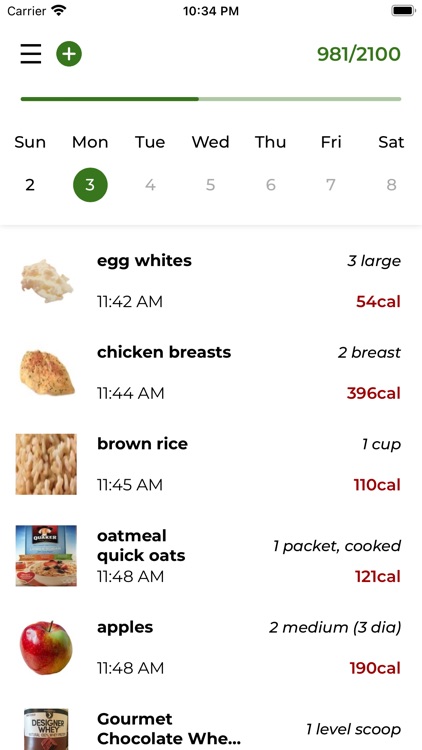The image appears to be a screenshot from an iPhone, showcasing a calendar or task management app with a focus on dietary tracking. At the top left corner, there's a three-line hamburger menu icon, next to which is a white plus sign within a green circle, indicating the option to add new items or tasks. In the upper right-hand corner, there is a progress indicator displaying "981/2100," which likely denotes completed tasks or goals out of a total target.

Below the progress indicator, the app lays out a week view starting from Sunday the 2nd to Saturday the 8th, with each weekday displayed horizontally. Monday the 3rd is highlighted in green, suggesting it is the selected day.

Further down, the app lists various grocery items accompanied by images, timestamps, quantities, and caloric information. The first entry is for egg whites, depicted with an image of fried egg whites. The entry details "Egg Whites" consumed at 11:42 AM, with a quantity of "three large" and 54 calories. The second entry is for a chicken breast, represented by an image of a cooked chicken breast, consumed at 11:44 AM, with a quantity of "two breasts" and 396 calories. Additional items on the list include brown rice, oatmeal (quick oats), apples, and gourmet chocolate whey protein, each with similar detailed information.